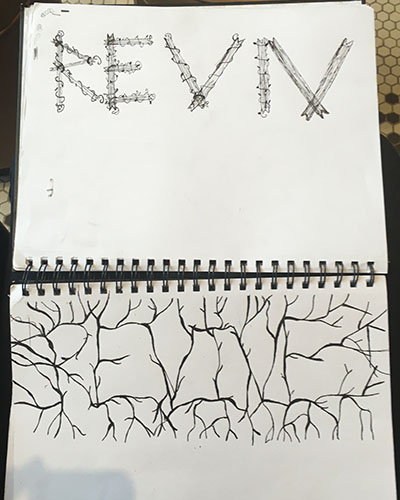In this image, we see an open sketchbook, with its spine running horizontally through the center of the frame. Both the top and bottom pages are completely blank, devoid of any lines or markings typically found in a college-ruled notebook. The pages feature drawings sketched in either pencil or pen. The drawing on the bottom page exhibits an abstract, flowing design reminiscent of tree branches, though it doesn’t seem to depict any specific object. Meanwhile, the top page contains the word "REVIX" drawn prominently in capital letters.